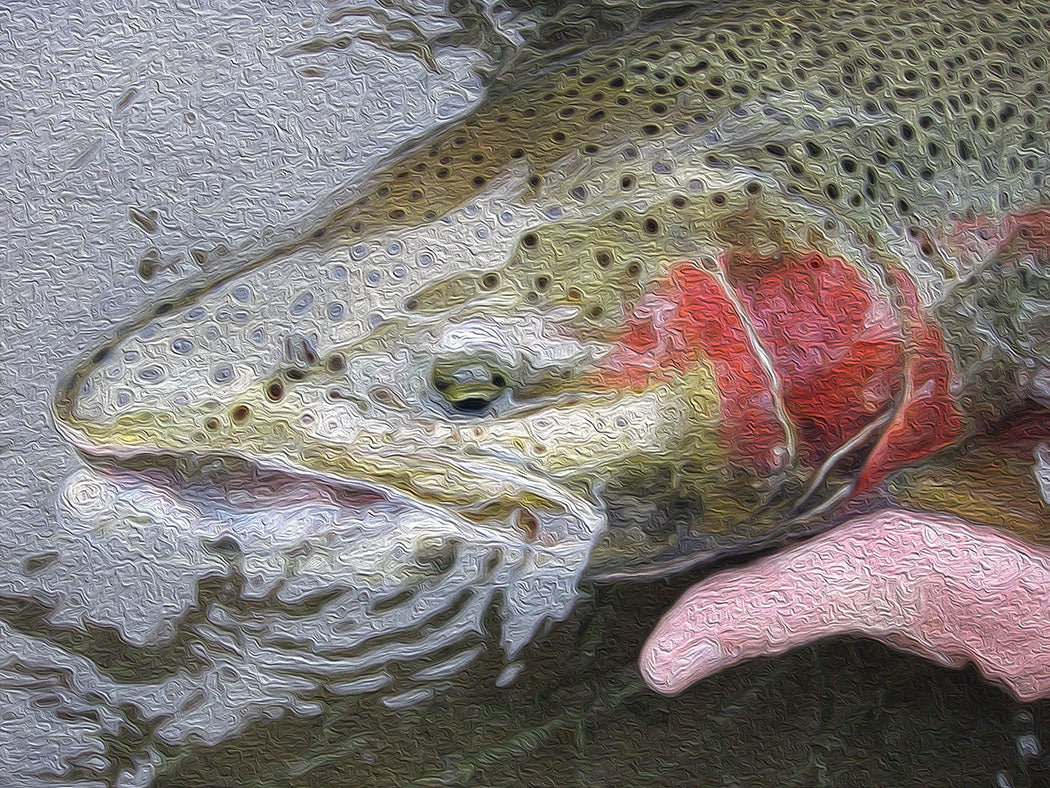The image depicts a large fish being held by a hand, which appears pink and emerges from the bottom right corner of the frame. The fish is characterized by a pointed nose, a flat head, and a large mouth akin to that of a large mouth bass. The fish's body features an array of black and brown dots on its back and scales that range in color from olive green to yellowish-brown, creating a muddled appearance. Around its gills, the fish exhibits pink and red hues, which streak toward its eye. The scene is filtered to introduce a ripple-like, wavy texture, giving the impression that both the fish and the hand are underwater, with light veins refracting off the fish's surface. This filtered effect adds an unsettling, painted quality to the photo, amplifying the sense of distortion and enhancing the overall surreal aesthetic.